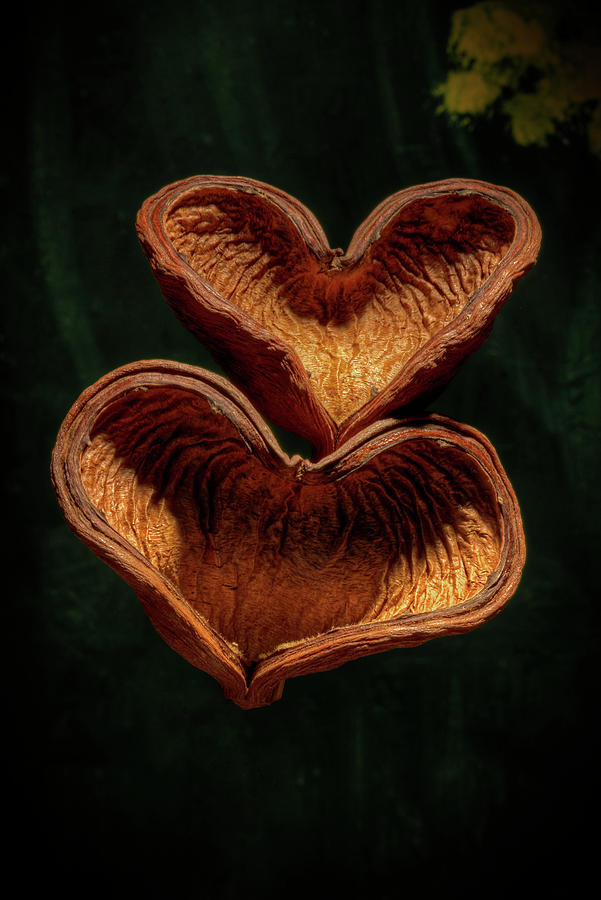This is a close-up, macro photograph of an opened walnut shell, uniquely shaped like two interlocking hearts, positioned against a predominantly dark background with streaks of green. The top heart is narrower and leans against one of the lobes of the larger, plumper heart below it. Both pieces have been hollowed out, revealing interiors that vary in shades of orange, burnt orange, gold, tan, and brown, with the top heart displaying more light inside. The exteriors are predominantly brown with red accents and an outline that resembles light orange, flame-like shading. Slight shadows enhance the three-dimensionality, with a notable shadow outlining another heart shape within the bottom piece. The intricate textures suggest a rough, ridged surface. A faintly visible tree appears in the right corner of the image, adding a subtle depth to the composition.